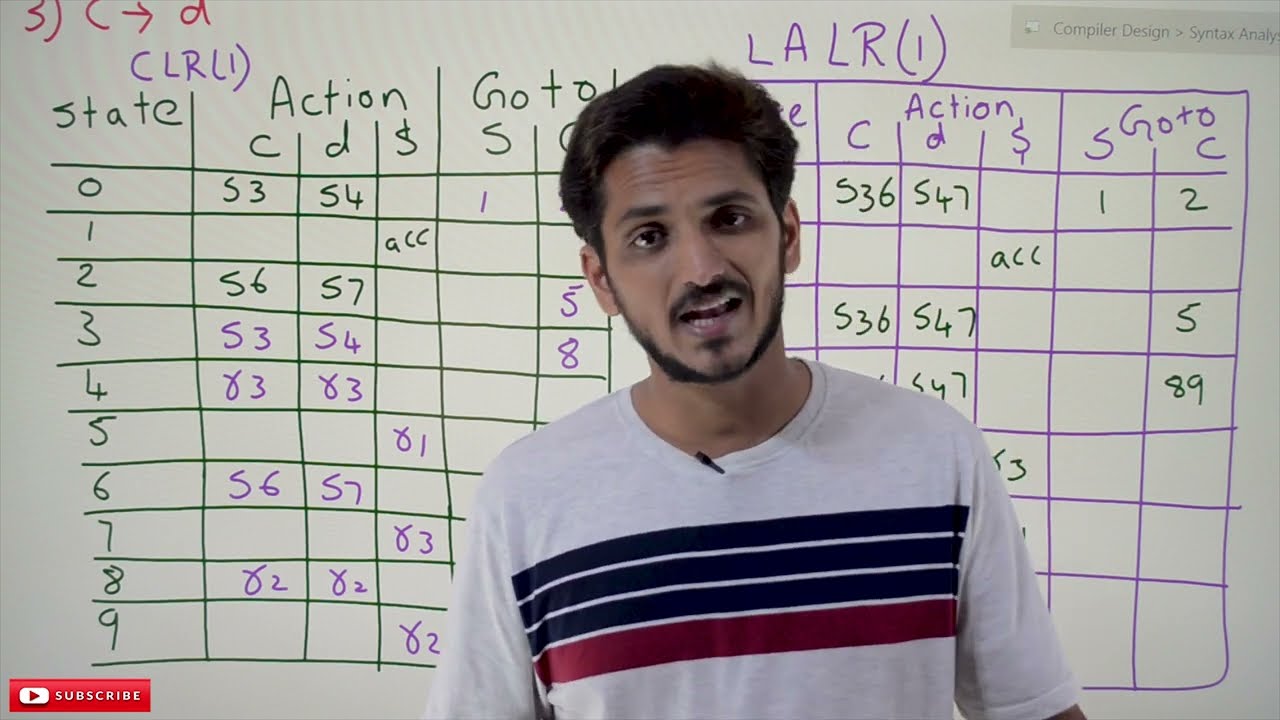In the image, a gentleman of Indian descent with a dark complexion and medium-cut black hair is standing in front of a detailed whiteboard, speaking with his mouth open. He sports a scraggly black beard and mustache and is dressed in a white t-shirt under a short-sleeved shirt that features three dark stripes and one prominent burgundy stripe across the chest. Additionally, he has a pen tucked into his collar. The whiteboard behind him is filled with an extensive array of information, including columns and rows labeled with data, numbers, and various headings. The most visible labels at the top include "State," "Action," and "CDS." The board appears to be an intricate action chart possibly related to "Computer Design Syntax Analysis" or a similar subject, as inferred from the text on the board. In the bottom left corner of the whiteboard, there's a red "Subscribe" button along with a YouTube arrow, set against the overall white background. The gentleman is partially obscuring some of the board's content, which adds to the complexity of the visual data presented.